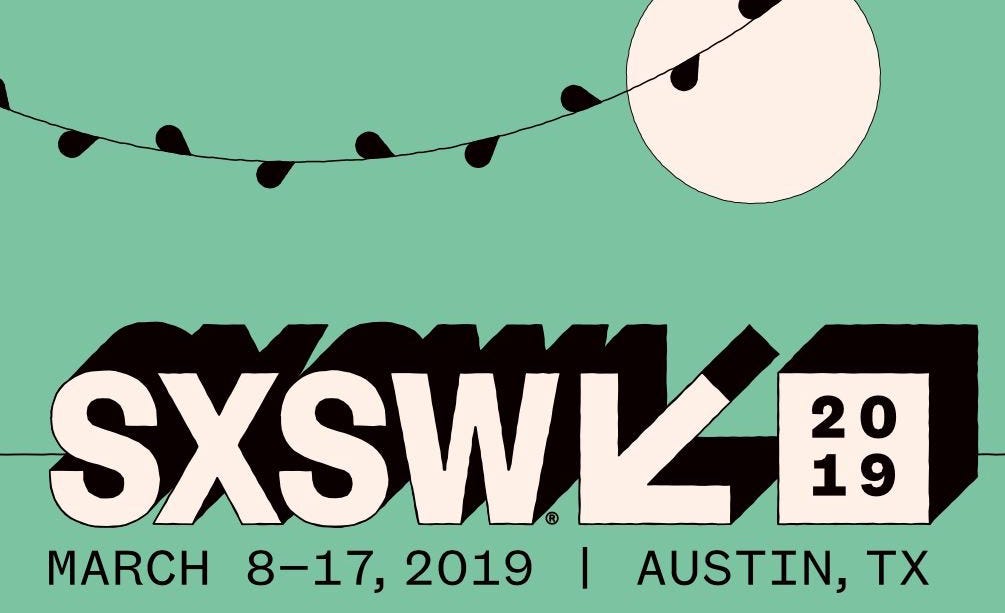This is a detailed promotional flyer for the renowned annual music festival, South by Southwest (SXSW), set against a soft turquoise-green background. The upper right corner features a moon, under which stretches a garland adorned with black decorative lights. Below this, the event's name, "SXSW", is prominently displayed in bold white letters with a black shadow effect, accompanied by a left-pointing arrow. The year "2019" is conspicuously placed beneath it, followed by the dates "March 8th to 17th, 2019" and the location "Austin, Texas" in a lighter black text.